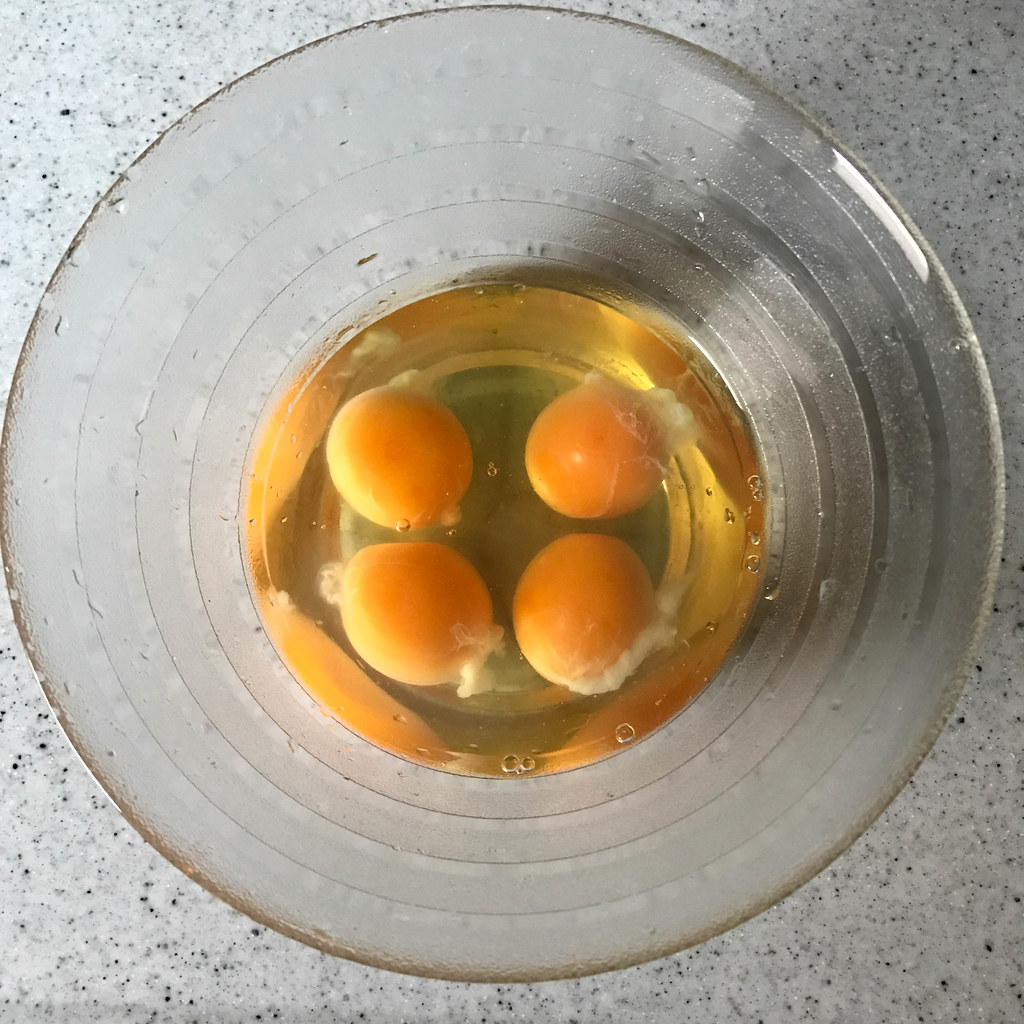A detailed description of the digital photograph taken indoors on a kitchen counter shows a marble countertop with characteristic black specks spanning the upper right, upper left, bottom right, and bottom left corners of the image. Central to the photograph is a large, clear bowl, likely made of glass or high-quality plastic, marked by rings that ascend from the base to the rim. In the bottom of the bowl, surrounded by a yellow liquid that may be vegetable oil, are four cracked eggs. These eggs are arranged in a 2x2 grid configuration, each with a prominent yellow yolk and some white surrounding it. A light reflection, possibly from sunlight or a camera flash, can be seen in the upper right of the photo.